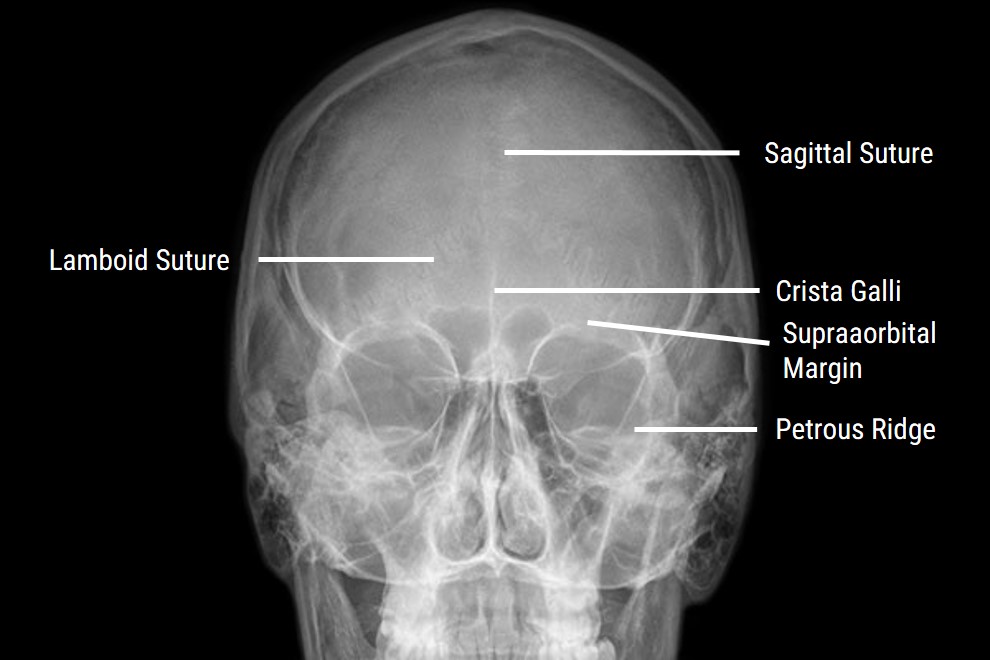This detailed black and white x-ray image of a human skull meticulously labels various anatomical features with white text and arrows. Key parts highlighted include the sagittal suture, lamboid suture, crista galli, suborbital margin, and petrous ridge. The image clearly shows the skull's structure, highlighting the intricate details of the teeth, nasal cavity, and eye sockets against a stark black background, emphasizing the labeled elements for educational purposes.